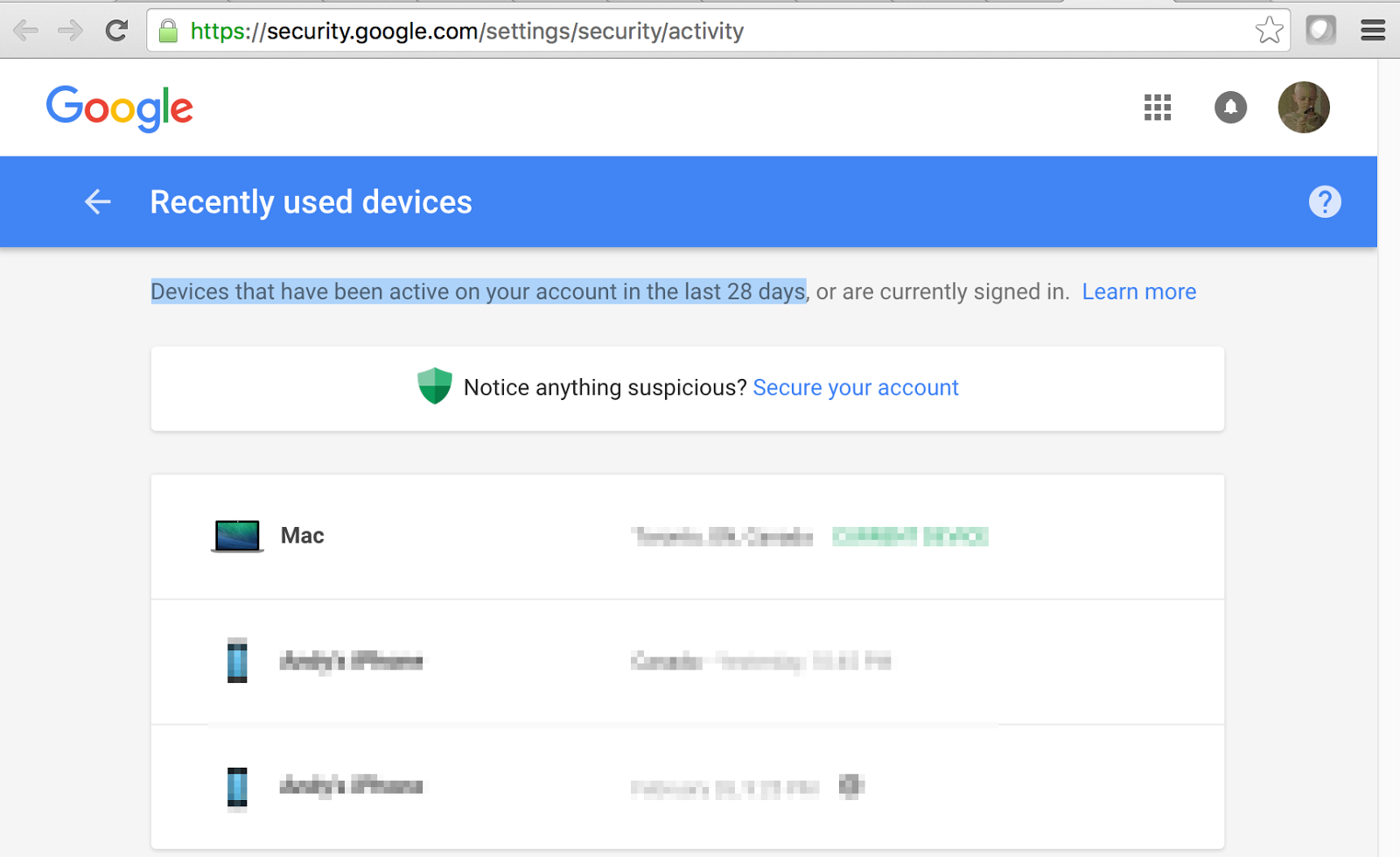This image is a screenshot of a webpage, likely from a Google account dashboard, displaying information about recently used devices. At the top of the page, a blue header with white text reads "Recently used devices," accompanied by a circular blue icon with a white question mark on the right side of the header. An arrow pointing to the left is situated next to the word "Recently."

Beneath the header, the background appears to be a mix of white and gray tones. A small blue notification box in black text reads, "Devices that have been active on your account in the last 28 days or are currently signed in." Notably, the phrase "or are currently signed in" is not part of the blue box.

Next to this notification, there is a "Learn more" link in blue text. Below, a wider white text box with black text states, "Notice anything suspicious?" followed by a blue link to "secure your account." Beside this text is a green icon resembling a shield or defender.

Further down, three more white text boxes list specific devices. The first box features an image of a laptop and reads "Mac," with additional details blurred out in black and green text. The second box shows a cell phone icon, possibly naming an iPhone registered to a particular user, though the specifics are also blurred. Similarly, the third box displays another cell phone icon, again with the device name and user details obscured.